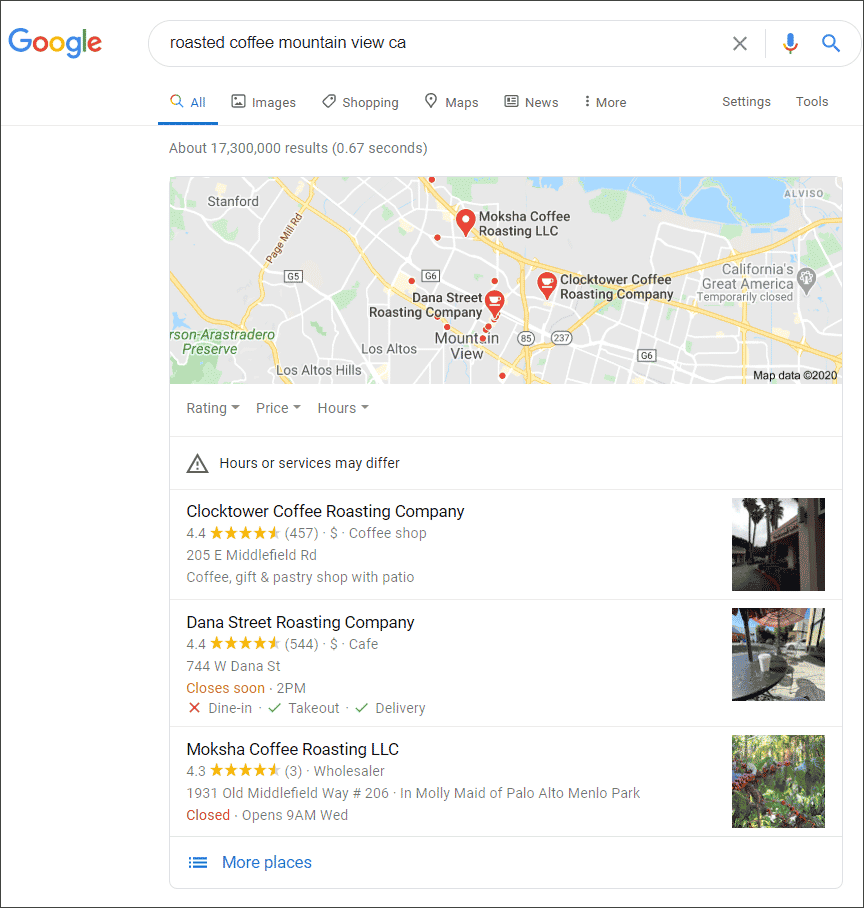This is a screenshot of a Google Search results page. The background is predominantly white, framed by black lines. In the upper left corner is the multicolored Google logo. To the right is the search field where the query "Roasted Coffee, Mountain View, California" has been entered. Adjacent to the search field on its right end are icons: a black X, a blue microphone, and a blue magnifying glass. Below the search field, there is a menu in gray font comprising options such as All, Images, Shopping, Maps, News, More, Settings, and Tools, with "All" being selected and highlighted by a blue underline. The search results display the text "About 17,300,000 results (0.67 seconds)" in gray font.

Below this, there is a small street map featuring three red arrows pointing to various coffee shops in Mountain View, California. Directly under the map, there are dropdown menus labeled "Rating," "Price," and "Hours" in gray font. A prominent alert box with a red rectangle and exclamation mark appears just below, stating "Hours or services may differ" in black font.

Further down, separated by a black line, is a listing with the bold black text "Cold Clock Tower, Coffee Roasting Company."